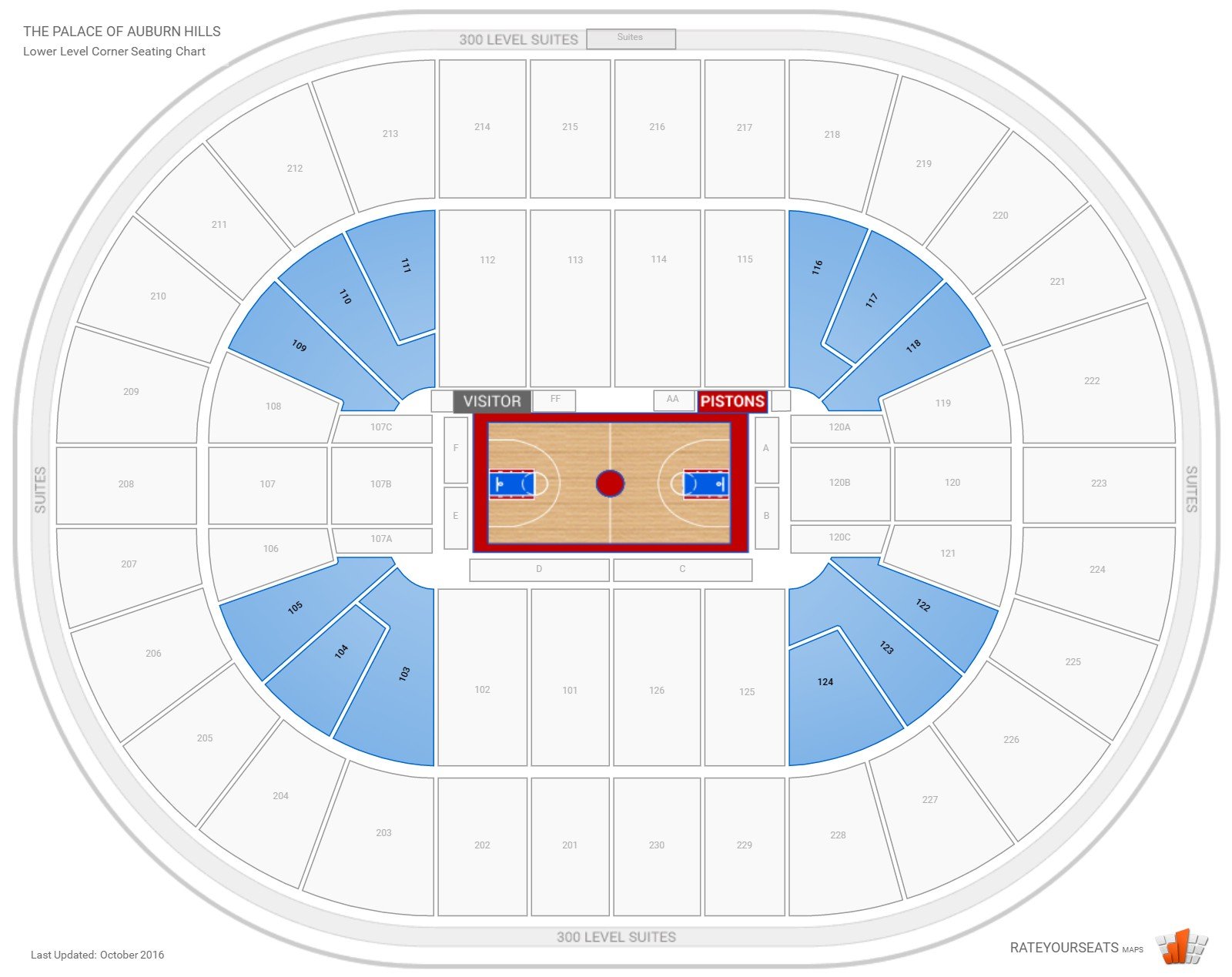A detailed layout image of the Palace of Auburn Hills basketball arena is presented, courtesy of rateyourseats.com. At the center of this detailed illustration is a basketball court, featuring a natural wood-colored floor with a prominent large circle in the middle. The keys near the baskets are distinctly painted in blue. The court is set within a large oval-shaped arena. The "Pistons" label is positioned on the right side of the court, while "Visitor" is on the opposing side. Surrounding the court are multiple sections of seating, depicted primarily in white with numerical labels indicating the separate sections. Certain corner areas of the seating are highlighted in blue, though the majority remain in white, suggesting no seats are currently selected or highlighted. The map does not show any seats as lit up or occupied. The image is a clean, organized representation of the seating arrangement and court design within the historic arena.